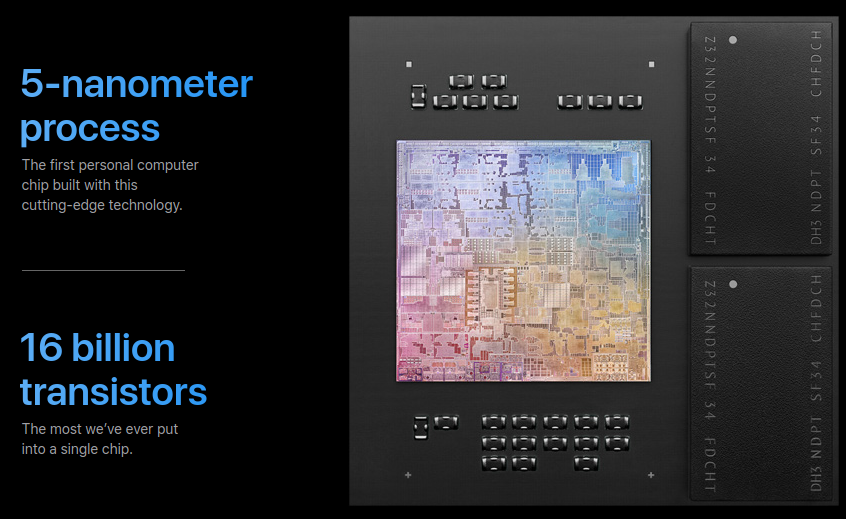The image features a horizontally oriented layout set against a black background. On the left side, blue text at the top reads "5-nanometer process." Beneath this in smaller white text is the description, "the first personal computer chip built with this cutting-edge technology." Continuing downward, another blue text section displays "16 billion transistors," followed by white text stating, "the most we've ever put into a single chip." The right side of the image showcases the intricate inner workings of the computer chip itself, displaying a vibrant array of colors including purple, blue, light yellow, and light blue. The chip is set within a dark gray panel, detailed with various microstructures and two vertical black rectangular components. Rows of small knobs are visible above and below the chip, illustrating its complex and detailed design, indicative of an advanced electronic device.